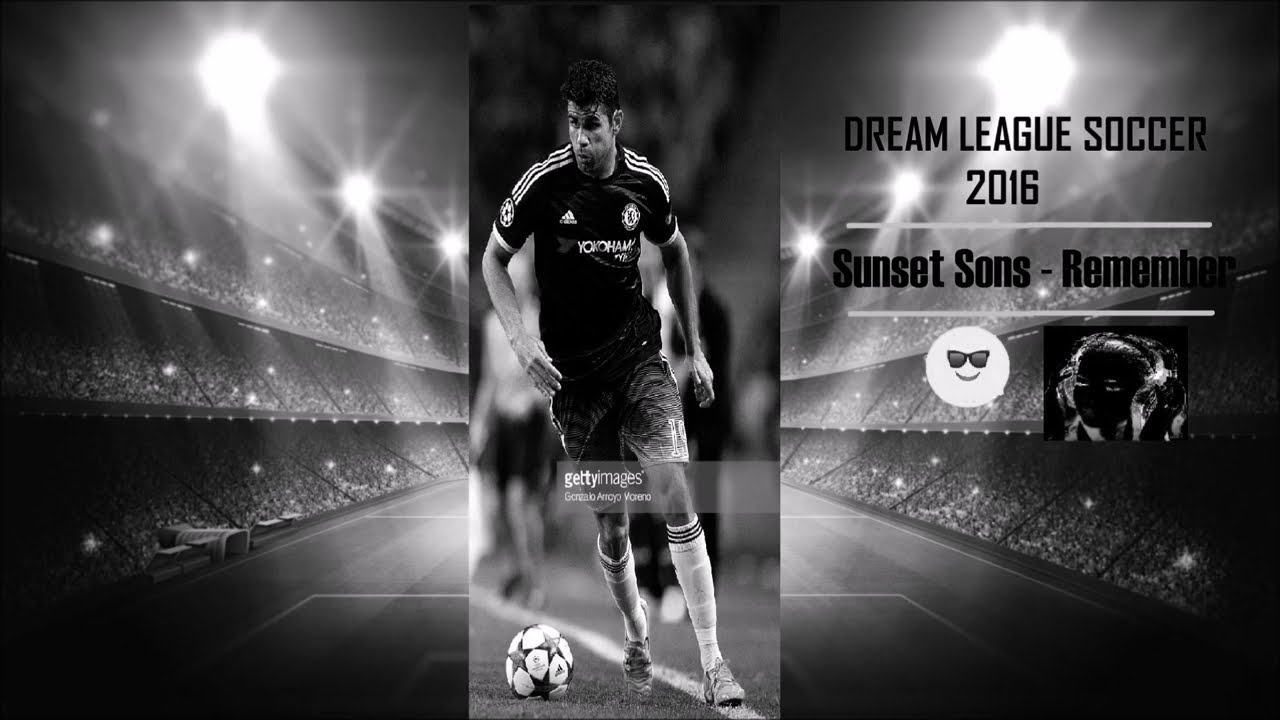This horizontal rectangular image is black and white and consists of three sections: a left and right section displaying a soccer stadium and a smaller center section showcasing a soccer player. The left panel shows a darkened, three-tiered stadium packed with spectators, with overhead lights visibly illuminating the field. The right panel mirrors this scene with the opposite side of the stadium. Both sections are slightly blurred, suggesting the intensity and focus of the central action.

In the center strip, under better lighting, is an image of a European soccer player. He has dark, likely sweaty hair and wears a jersey with distinctive Adidas branding and stripes on the shoulders, complemented by black athletic shorts and knee-high white socks with three stripes at the top. His body faces forward with a slight twist to the right, while his head turns a bit to the left, capturing a dynamic moment as he runs toward a soccer ball adorned with black and gray stars, positioned just to his left foot, indicating he is about to kick it.

Above the player, in the right panel, bold black capital letters announce "Dream League Soccer 2016," followed by "Sunset Suns-Remember." Below this text is a playful image of a sun with a smiley face and sunglasses. The background highlights blurred figures and additional sections of the stadium, encapsulating the energy and atmosphere of a live soccer match.